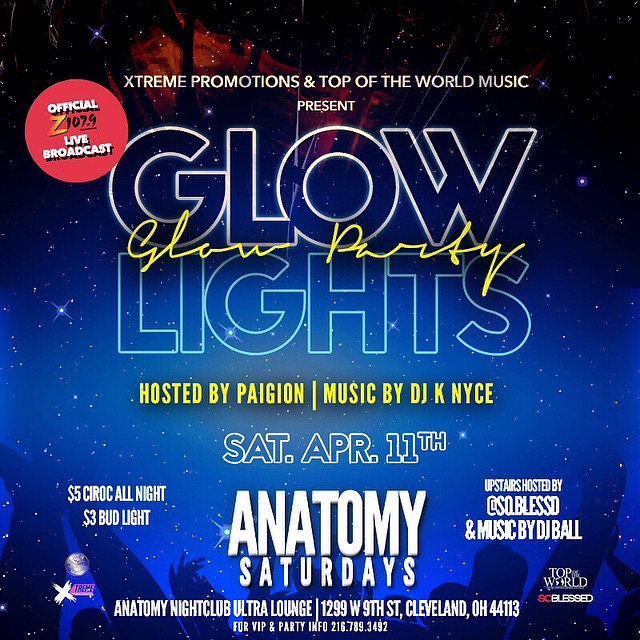**Extreme Promotions and Top of the World Music present: Glow Lights Glow Party**

Beneath a captivating night sky filled with shining stars in a gradient from darkest blue to a lighter hue, this vibrant flyer announces an electrifying event. At the top, in bold white capital letters, it reads "EXTREME PRODUCTIONS AND TOP OF THE WORLD MUSIC PRESENT." Dominating the center, the words "GLOW LIGHTS" appear in large, translucent letters outlined in white, with "Glow Party" in whimsical yellow cursive nestled in between. 

On the upper left corner, a small red circle contains "Z 107.9" with a lightning-like orange "Z," announcing an "Official Z 107.9 Live Broadcast" written in white. Prominently, it highlights "HOSTED BY PAGEAN" and "MUSIC BY DJ K NICE," both in yellow capital letters. 

Further details include:
- Date: SATURDAY, APRIL 11th
- Event Name: ANATOMY SATURDAYS written larger, with "Anatomy Saturdays" in capital white letters underneath.
- Venue: Anatomy Nightclub Ultra Lounge, 1299 W 9th Street, Cleveland, Ohio 44113.

Additional offerings such as "$5 Ciroc All Night" and "$3 Bud Light" are noted in the lower left, while the right side mentions "Upstairs hosted by @SoBlessed" with music by "DJ Ball."

The footer provides contact information for VIP and party details: 216-789-3492. Silhouettes of dancers and excited guests fill the bottom of the design, enhancing the festive and dynamic atmosphere of the advertisement.